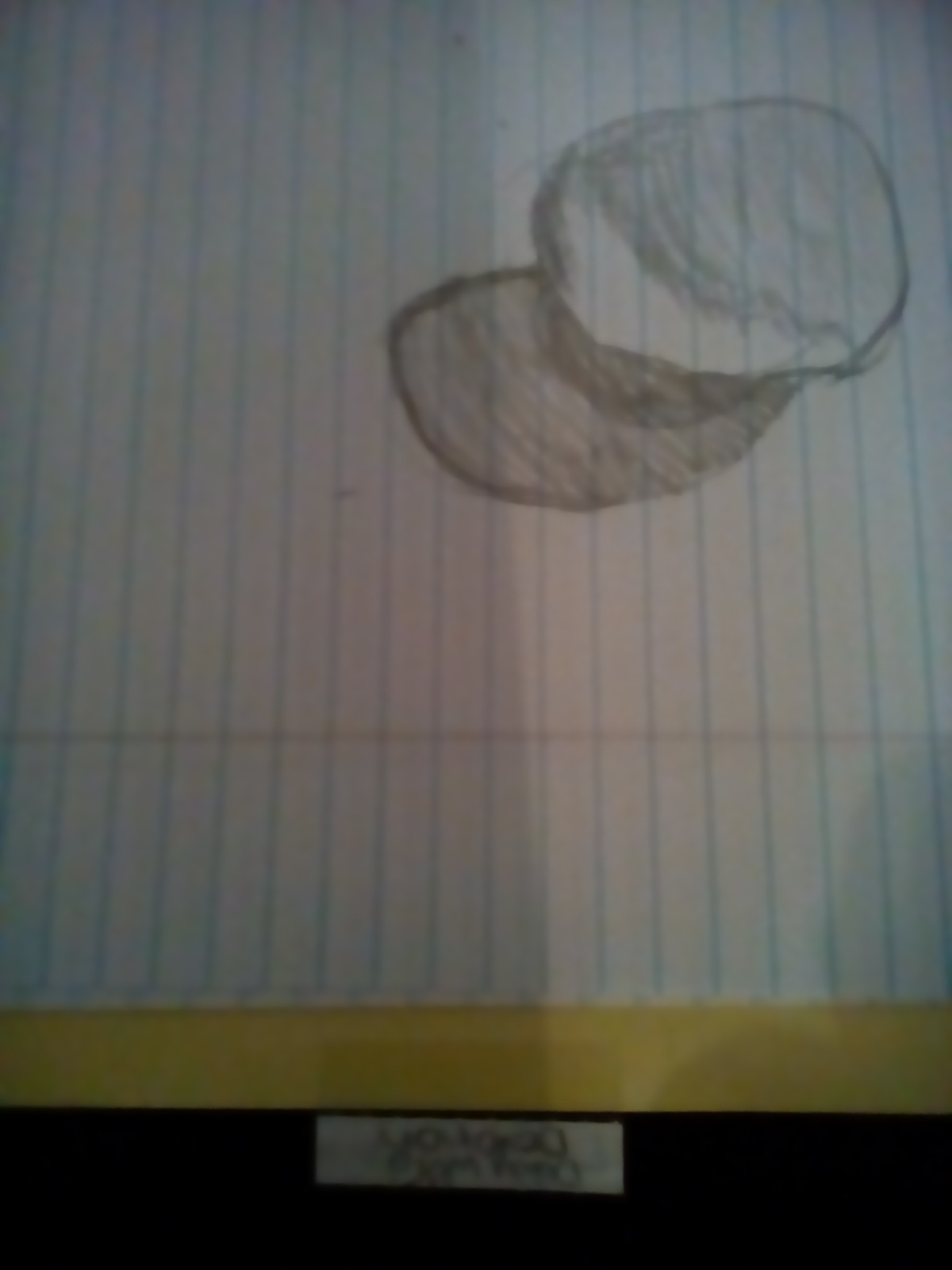This is a detailed, up-close photograph captured in portrait orientation. The main focus is a rectangular piece of notepad paper, slightly tilted to its side. On the upper right corner of the notepad, there is a simple drawing of a hat, complete with a brim and the crown of the hat. This notepad paper rests on a bright yellow sheet of paper, creating a vivid contrast in the background. Towards the bottom of the image, a label appears, although the text is illegible. This label is positioned against a black bar that spans across the lower portion of the photo, adding a sense of structure to the composition.